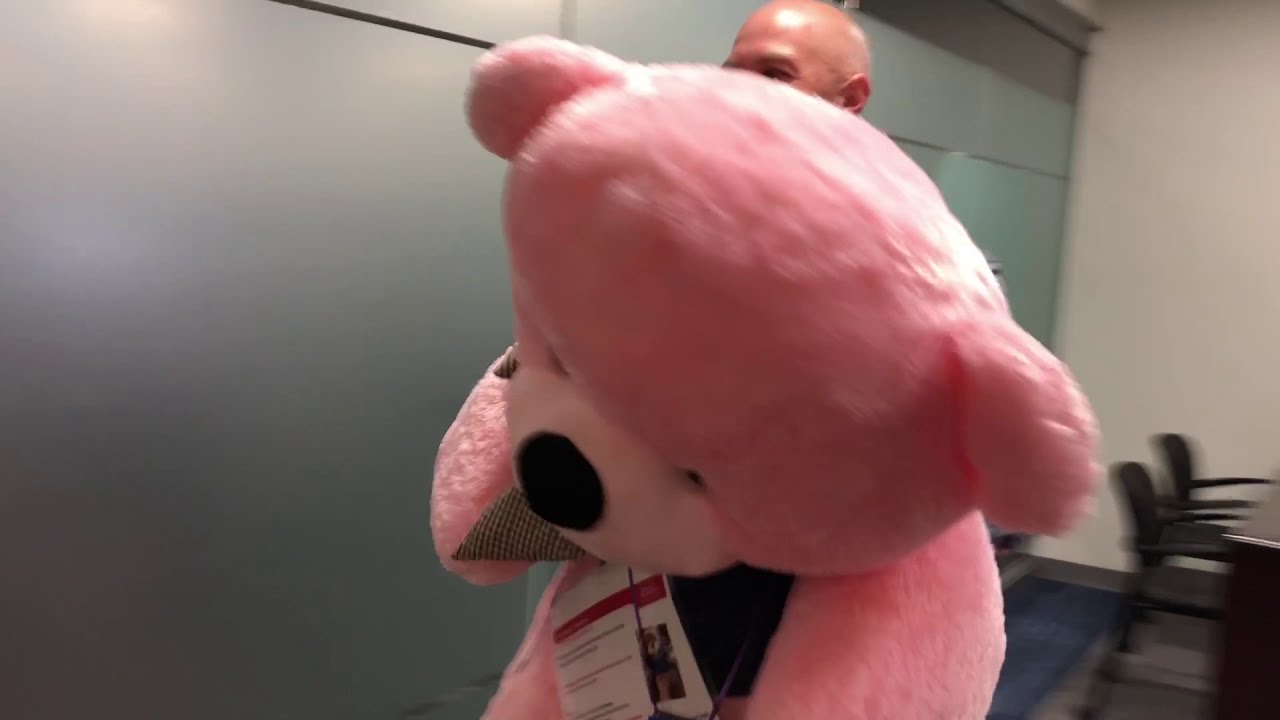The photograph depicts a life-sized, pink teddy bear being carried by a bald Caucasian man, whose head is the only visible part of him above the teddy bear. The teddy bear, which is so large it covers most of the man's face, has lighter pink snout, black eyes, and a prominent black nose. It appears to be new, with a white tag or booklet hanging around its neck. The bear also seems to be wearing a black vest or accessory. The setting appears to be an office, distinguished by a plain gray wall, some chairs at a desk, and frosted glass in the background. There are green shelves or cupboards along with a white wall situated to the left, and a dark-colored desk on the right. Despite the various background elements, the central focus remains on the enormous pink teddy bear, which looks like a thoughtful gift.